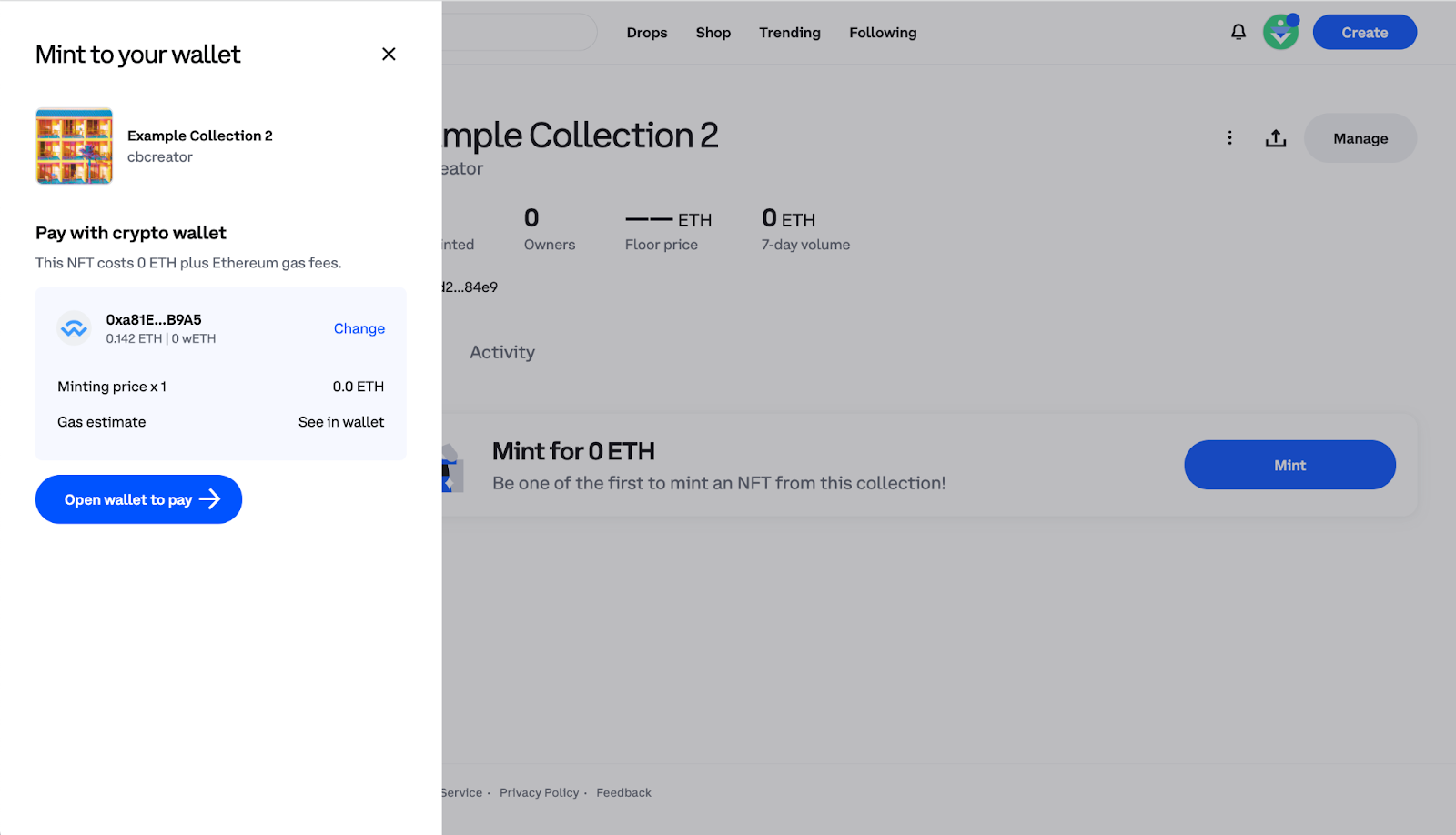The image features a light gray vertical rectangle centered on the screen, with a vertical rectangular white section on its left. At the top of the white section, bold black text reads "Mint to your wallet" with an X mark next to it. Below this, there's a small icon, followed by the bold text "Example Collection Two." Directly underneath, another bold text says "Pay with Crypto Wallet." Smaller, unreadable text follows, and towards the bottom lies a blue horizontal rectangle with white text that reads "Open Wallet to Pay" and an arrow pointing to the right.

Adjacent to this, in the gray section that is partially cut off on the left side, the text begins with "AMPLE Collection Two." It's as if the gray section is a magnified portion of the white part. Beneath this, some unreadable statistics are displayed. Near the bottom, the bold text "Mint for 0 ETH" is prominent, followed by lighter gray text stating, "Be one of the first to mint an NFT from this collection." The top right corner features a blue horizontal oval with the word "Create" inside it. Finally, opposite the "Mint for 0 ETH" text, there's a blue horizontal oval button with "Mint" written in white.